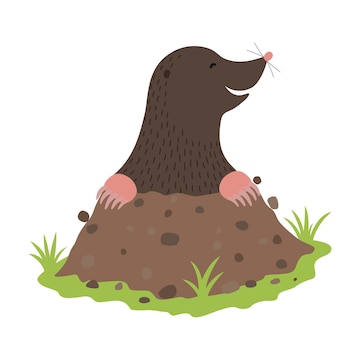This is a traditional-style cartoon of a cute and pleasant mole emerging from a dirt mound surrounded by grass. The dark brown mole, with his torso and paws visible above the dirt, faces to the right and smiles so hard that his eyes are closed. His small, pink nose adorned with two whiskers on each side stands out on his cheerful face. An ear hole is visible on the side of his head. His peach-colored paws and feet peek out from the lighter brown dirt pile, which is dotted with darker clumps. The mound of dirt is circled by green grass tufts, set against a plain white background, giving the image a simplistic and old-fashioned comic appearance suitable for a school child's drawing.